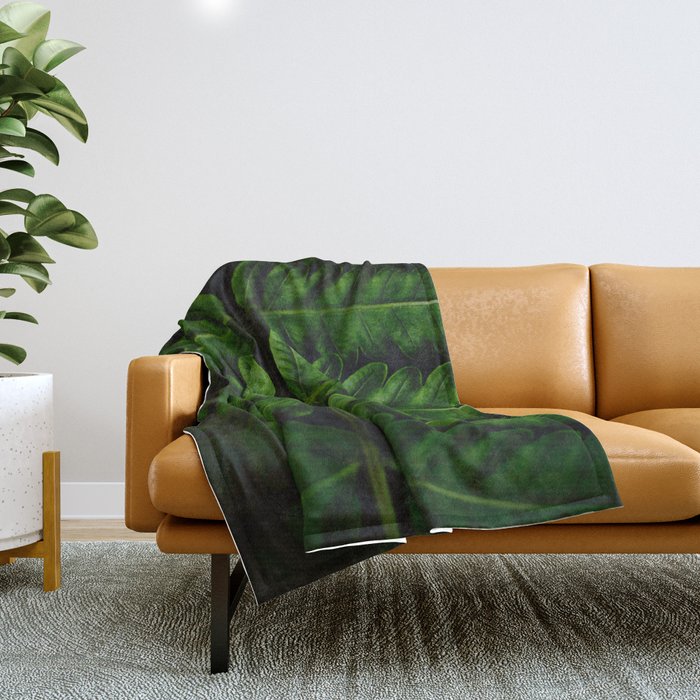This professional stock photograph captures a stylish living room scene with a prominent focus on a modern brown leather couch, which has an orange or terracotta hue. Draped over the backrest and left arm of the couch is a dark green blanket featuring a detailed botanical print of plant leaves and branches. The couch stands on dark brown legs and rests upon a light gray shaggy carpet. To the left of the couch is a white planter with a slender tall green indoor plant, placed in a cubic white pot with a wooden leg stand. The backdrop of the scene is a light gray wall with white trim, further accentuating the contemporary aesthetic of the room.